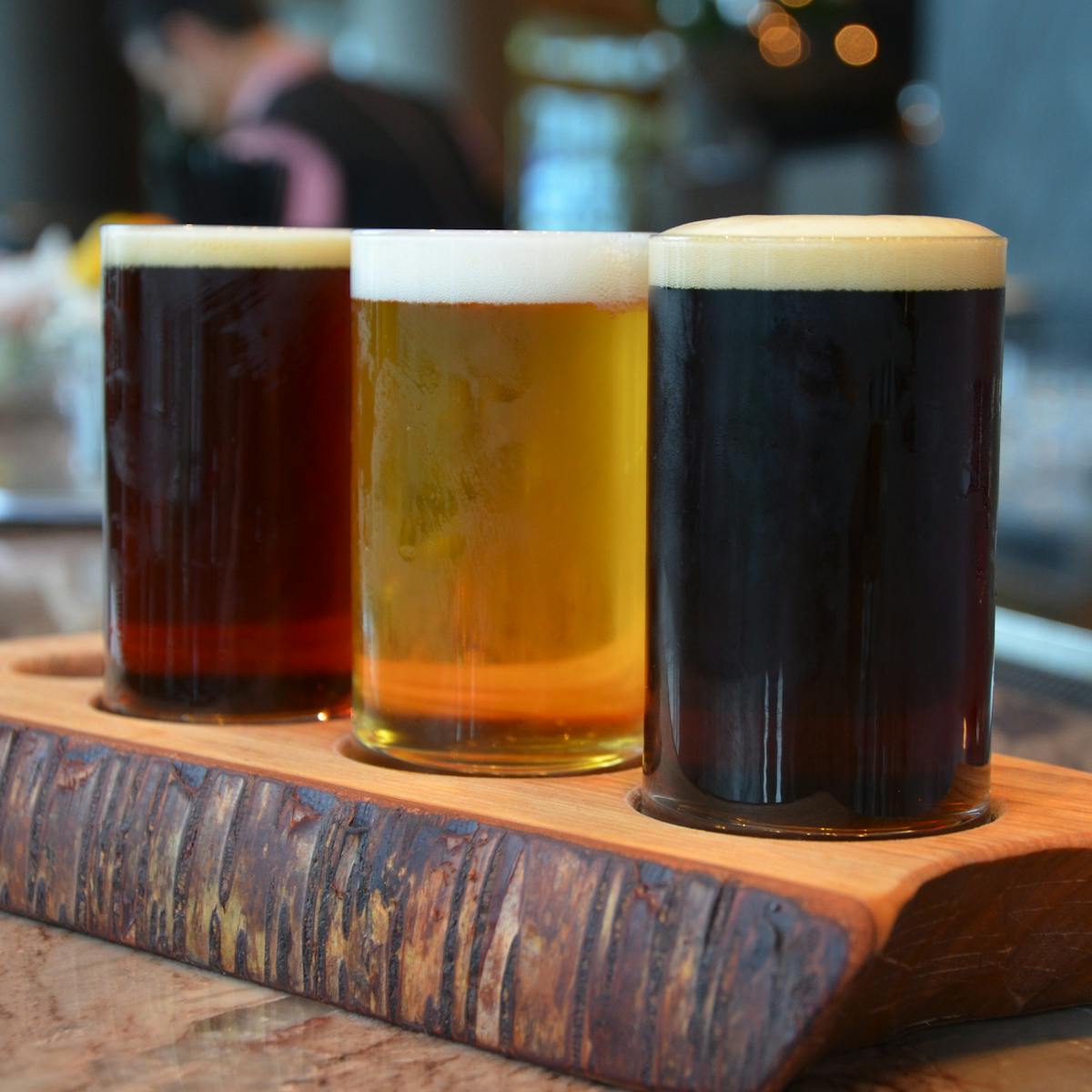This large square close-up photograph showcases a trio of beer mugs presented as a flight on a wooden serving board. The board features three cut-out circles perfectly fitting each mug, lined up diagonally from left to right. Each beer is distinct in color and has a frothy white head on top. Starting from the left, the beer is an amber hue, possibly a red or amber ale with a moderate foam cap. The center mug holds a golden beer, likely a pilsner or lager, with a thicker layer of foam. On the right is the darkest beer, an almost black stout, also topped with a foamy head. The wooden serving board rests on a countertop, which appears to be brownish granite, adding to the rustic aesthetic with its natural, tree-bark-like siding. Although the background is blurred, it hints at a busy restaurant or bar scene, including the faint outline of a man in dark clothing and soft, ambient lighting.